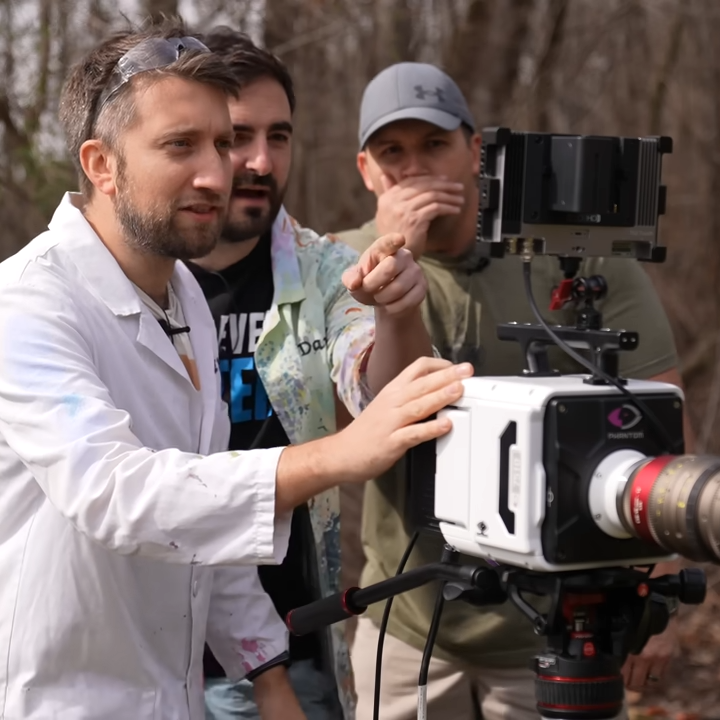In this outdoor image, three men are prominently positioned in the center, all gazing off to the right. The scene is set against a backdrop of trees and a bit of the sky, indicating a daytime setting. One of the men is wearing a white lab coat, giving him a distinguished appearance. The other two men are dressed more casually; one in an open button-down shirt layered over a T-shirt, and the other in a polo shirt paired with a baseball cap. In front of them stands a professional-looking camera mounted on a stand, with a white casing. The scene suggests they might be on a movie set, given their focused attention on the camera and the professional atmosphere. The color palette of the image includes various hues such as brown, white, tan, black, green, blue, red, gold, and silver. There is no visible text in the image.